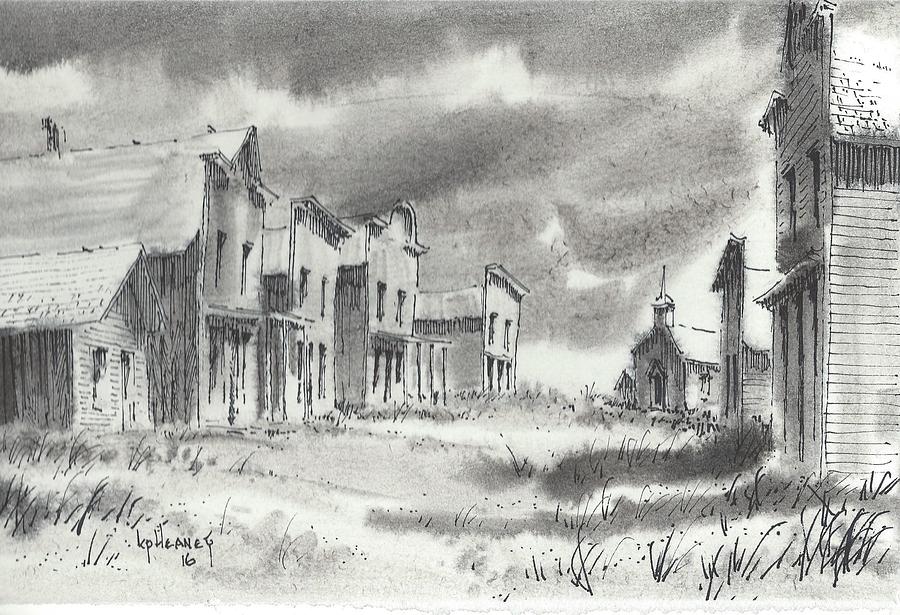This black and white image is a meticulously detailed, hand-drawn sketch, likely executed with a ballpoint pen or pencil. The artist, identified as KP Heaney, has signed the artwork at the bottom left corner, accompanied by the number 16. The composition invites the viewer to look down a path flanked by grassy areas, leading through a quaint village-like setting. On either side of the path, diverse houses and buildings rise, their architectural style reminiscent of the historic California missions and traditional Mexican influences from the pre-settlement era of California.

At the far right end of the path, a church stands prominently, adding a focal point to the scenery. The sky above is laden with clouds, casting a gloomy ambiance over the scene. The artist has employed a highly detailed approach, particularly focusing on the interplay of light and shadow to render depth and mood in the drawing. This technique of shadowing is executed with remarkable skill, enhancing the overall impact and emotive quality of the artwork.